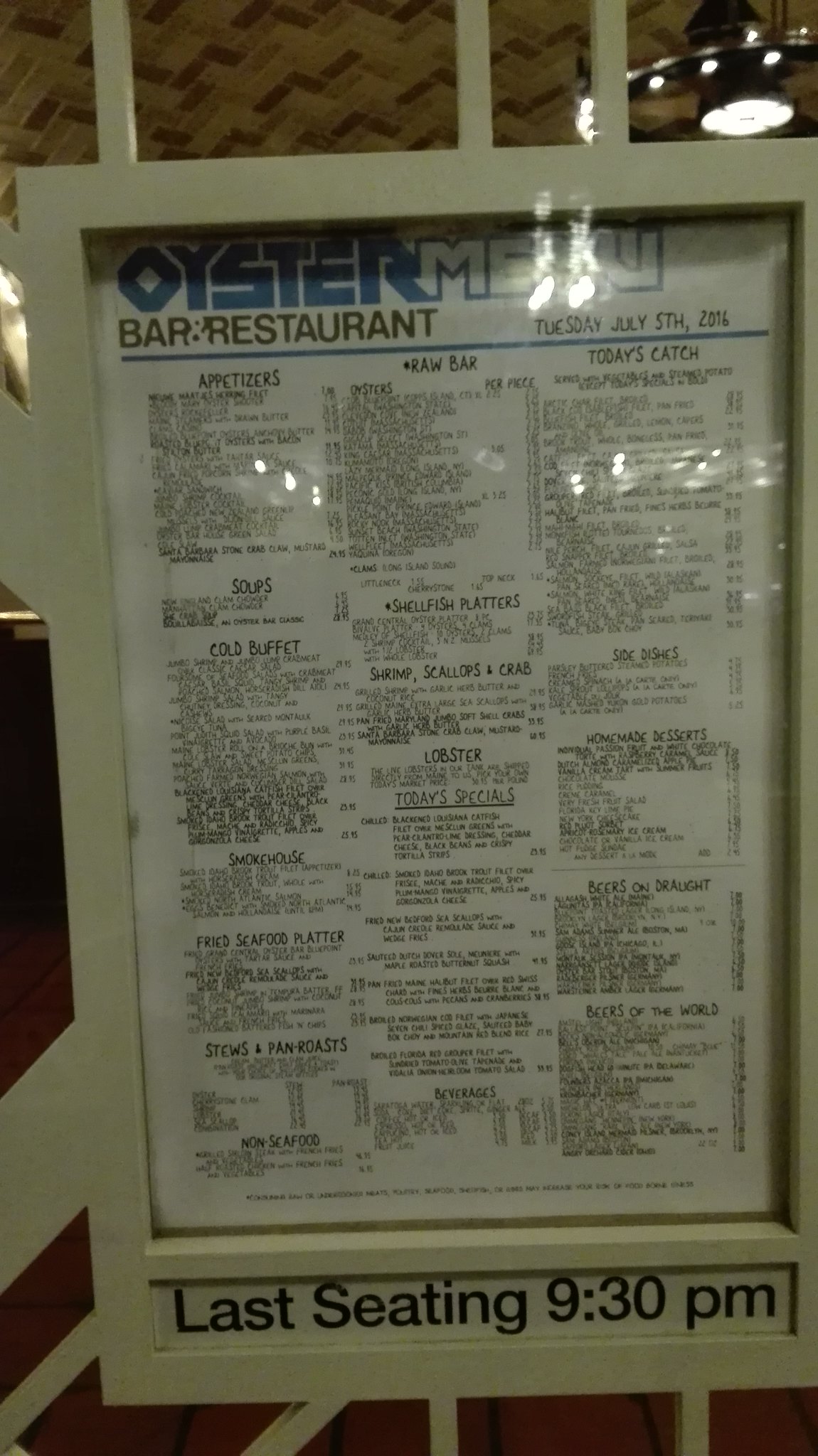Photograph of the Oyster Bar Restaurant menu, dated Tuesday, July 5th, 2016. The menu is predominantly handwritten, featuring a wide array of options:

- **Appetizers**
- **Soups**
- **Cold Buffet**
- **Smokehouse**
- **Fried Seafood Platter**
- **Stews and Pan Roasts**
- **Non-Seafood Dishes**
- **Raw Bar**
- **Shellfish Platters**
- **Shrimp**
- **Scallops and Crab**
- **Lobster**
- **Today's Specials**
- **Beverages**
- **Today's Catch**
- **Side Dishes**
- **Homemade Desserts**
- **Beers on Draft**
- **Beers of the World**

Notably, the menu indicates that the last seating is at 9:30 PM.